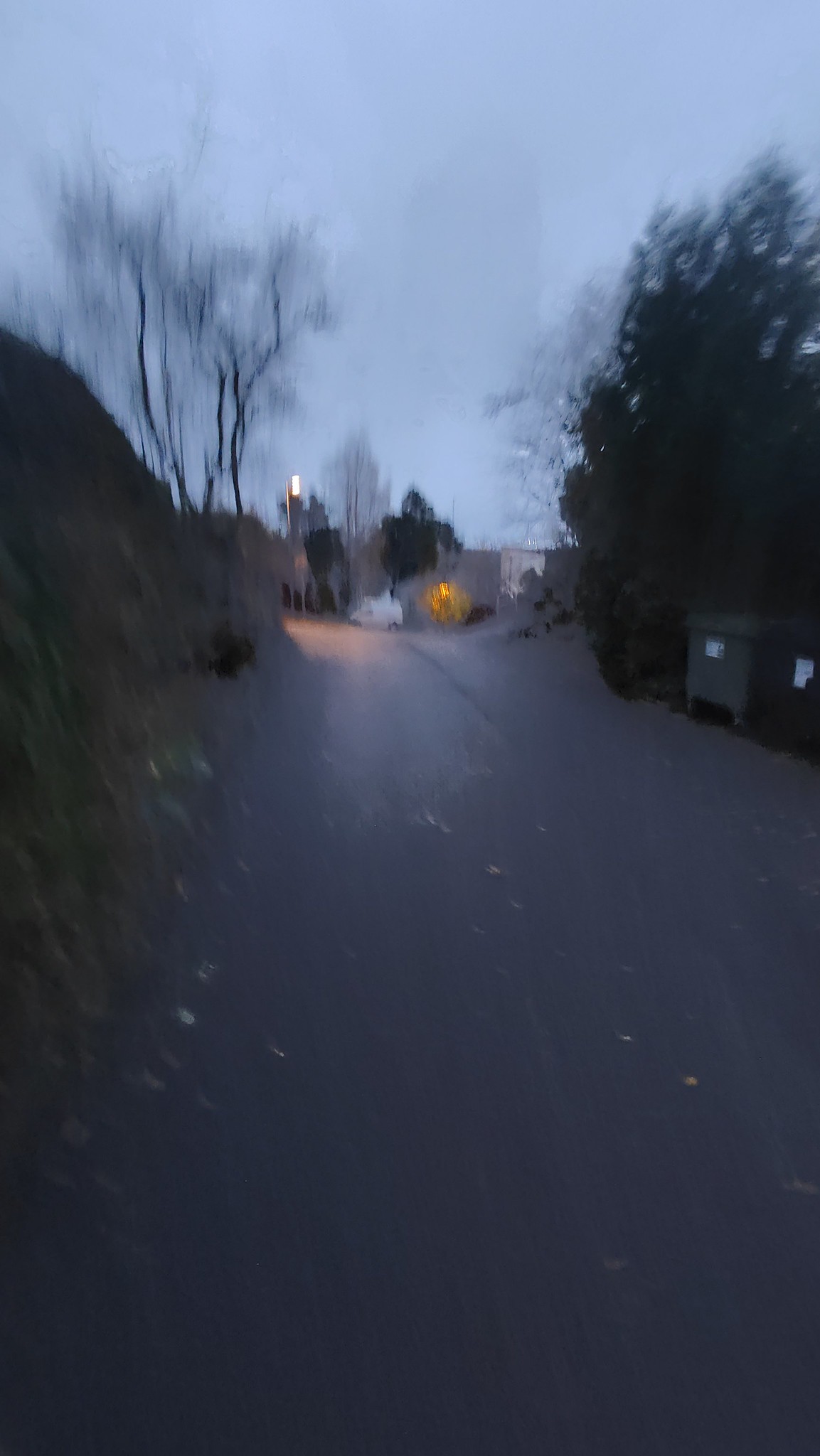In this blurry evening or possibly nighttime scene, the sky appears cloudy, casting a grayish hue over the landscape. The focal point is a narrow driveway or back alley that stretches into the distance, ending at what seems to be a building surrounded by various trees. A street lamp near the end of the driveway emits a yellow glow, illuminating patches of the ground. Towards the bottom of the image, where the light doesn’t reach, the scene is much darker.

On the left side, a green hill rises with several dead, tall, thin trees positioned in front of it. A green dumpster is also visible to the right of these trees. Further left, there are more thick, bushy trees. The right side of the driveway is lined with similar dense trees and another large garbage bin, resembling a city dumpster.

There is a parked white vehicle, possibly a car or truck, in the background near the end of the driveway, adding to the suburban feel of the scene. The moisture on the camera lens and blurriness of the image create an additional layer of obscurity, making it challenging to discern finer details. However, the presence of a faint figure walking adds a touch of life to this otherwise quiet, misty scene.